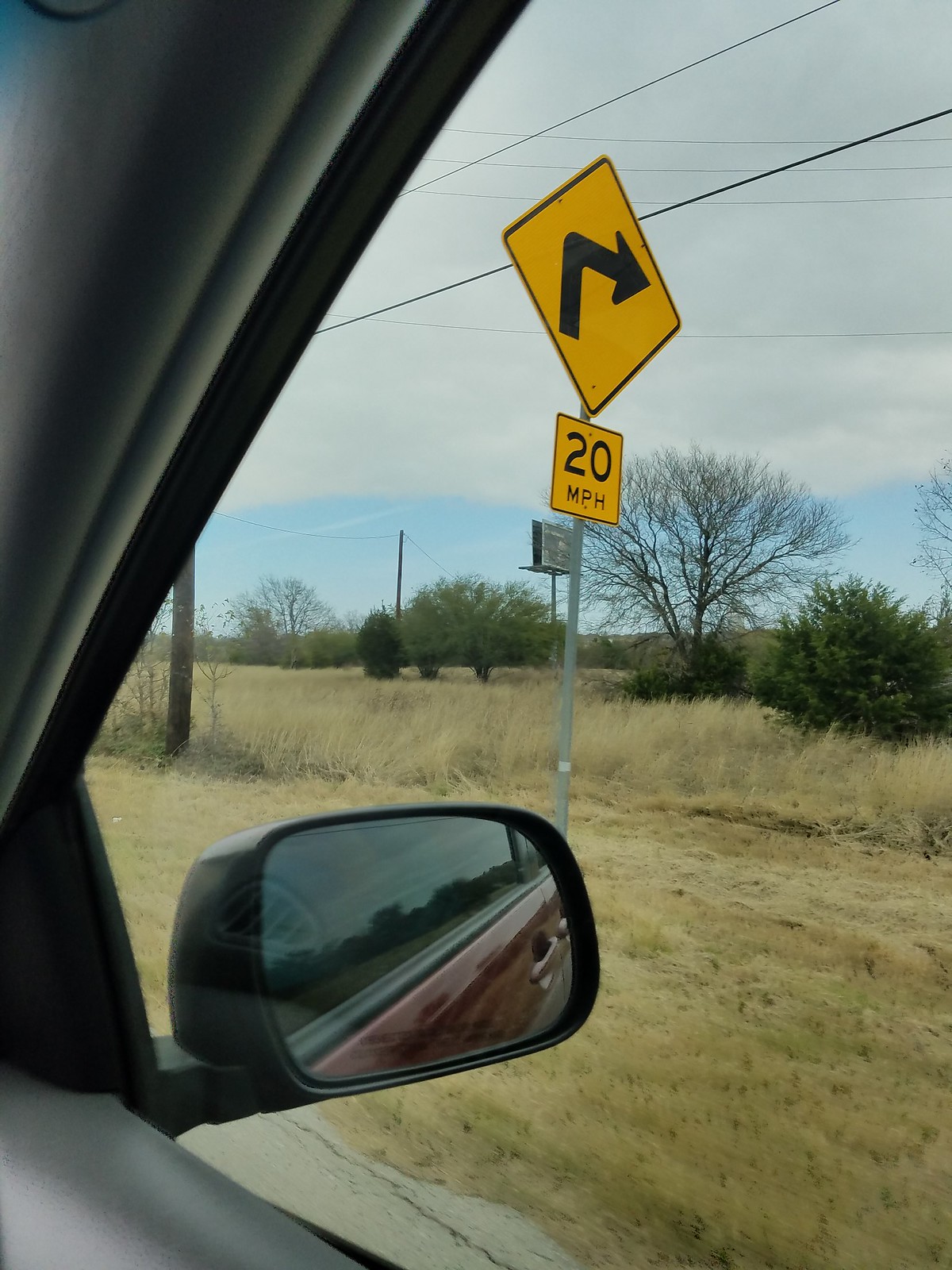This image, captured from inside a vehicle, features a dynamic view of the sky and roadside signage. The upper portion of the sky is a pristine white, transitioning into a gentle light blue towards the bottom. Centrally positioned are two road signs attached to a single gray pole. The top sign is diamond-shaped with a bold black border and a vibrant yellow background, featuring a black arrow pointing to the right. Directly below it resides a square-shaped yellow sign that prominently displays "20 MPH" in black text. Completing the scene, the car's mirror is visible at the bottom edge of the image, framing the perspective from the vehicle.